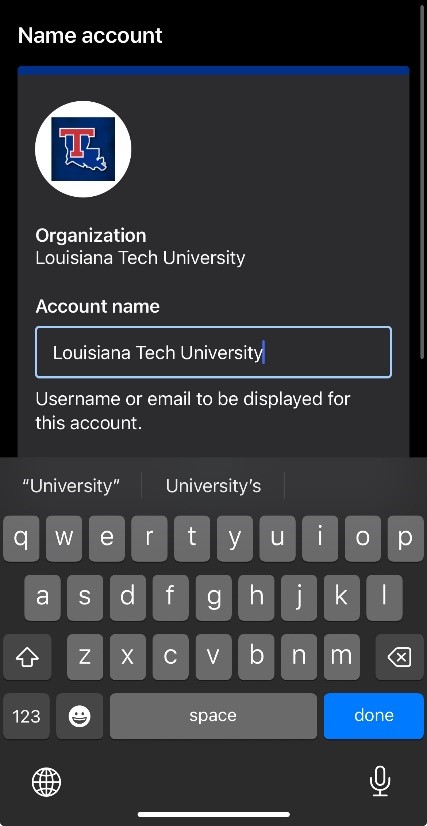The image displays a smartphone screen showcasing a form for creating or managing an account, likely for Louisiana Tech University. The top section of the screen features the text "NAME" and "ACCOUNT" in white, situated on a black background in the upper left corner. Below this, there is a rectangular section, with a blue strip at the top and a gray background.

On the left side of the screen, inside a white circle, there is a stylized outline of the state of Texas in blue, bordered in white. Enclosed within the outline is a large red "T," possibly representing "Texas" or "Tech." Just below this icon, in white, it says "Louisiana Tech University."

Further down the screen, bold white text spells out "ACCOUNT" with each letter capitalized. Below the account information, a form field appears, outlined in light blue on a gray background. Inside this field, "Louisiana Tech University" has been entered.

Underneath the form field, the text prompts "Username or email to be displayed for this account." Above the on-screen keyboard, there are suggestions such as "university" in quotation marks and "universities'" with an apostrophe.

The keyboard itself features gray keys with white letters. The layout includes the standard QWERTY arrangement: the first row has Q-W-E-R-T-Y-U-I-O-P, the second row A-S-D-F-G-H-J-K-L, and the third row Z-X-C-V-B-N-M. The space bar shares the same gray color, and to its right, a blue button with the word "Done" is visible.